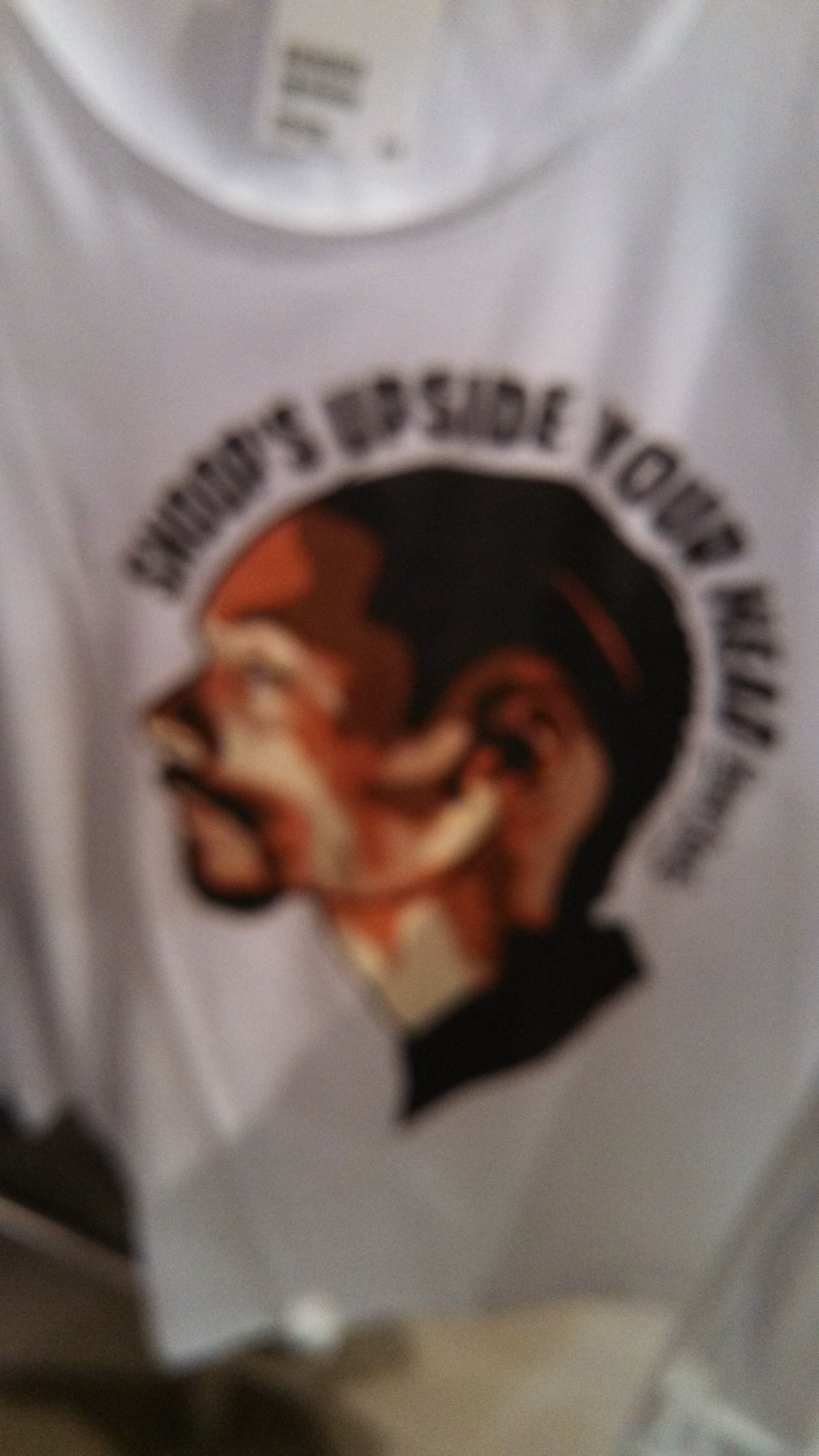A blurry image captures an oversized white T-shirt displayed in a store. The focus is so poor that the black font on the collar's tag is unreadable. Dominating the shirt's front is a cartoon side profile of Snoop Dogg facing left. He is depicted from the neck up, wearing a black shirt. Encircling his head are partially readable words, including "Snoop's Upside Tour," with additional, indistinguishable text due to the blurriness. The font is standard and black, blending with the overall design of the T-shirt.